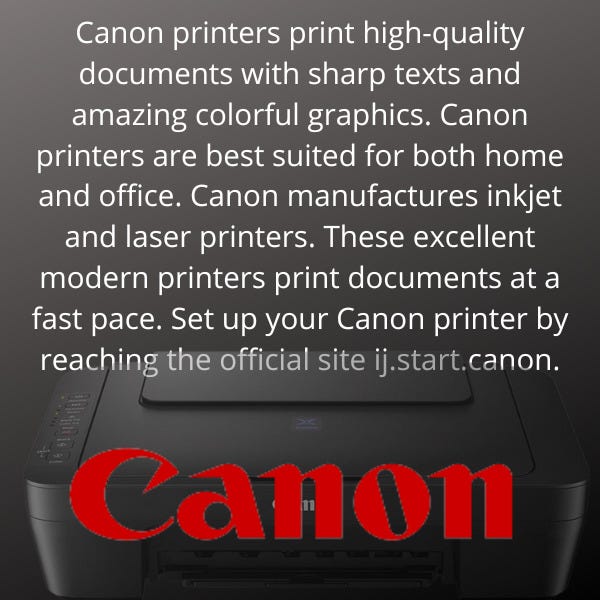The image is an advertisement for Canon printers, set against a dark gray background. Dominating the foreground is a high-resolution picture of a Canon printer, with the word "Canon" prominently written in bright red at the bottom, making it stand out dramatically. The detailed text on the image emphasizes the superior quality of Canon printers, stating: "Canon printers print high-quality documents with sharp text and amazing, colorful graphics. Canon printers are best suited for both home and office. Canon manufactures inkjet and laser printers. These excellent, modern printers print documents at a fast pace. Set up your Canon printer by reaching the official site, ij.start.canon." This ad effectively highlights the efficiency, versatility, and reliability of Canon printers for varied use.